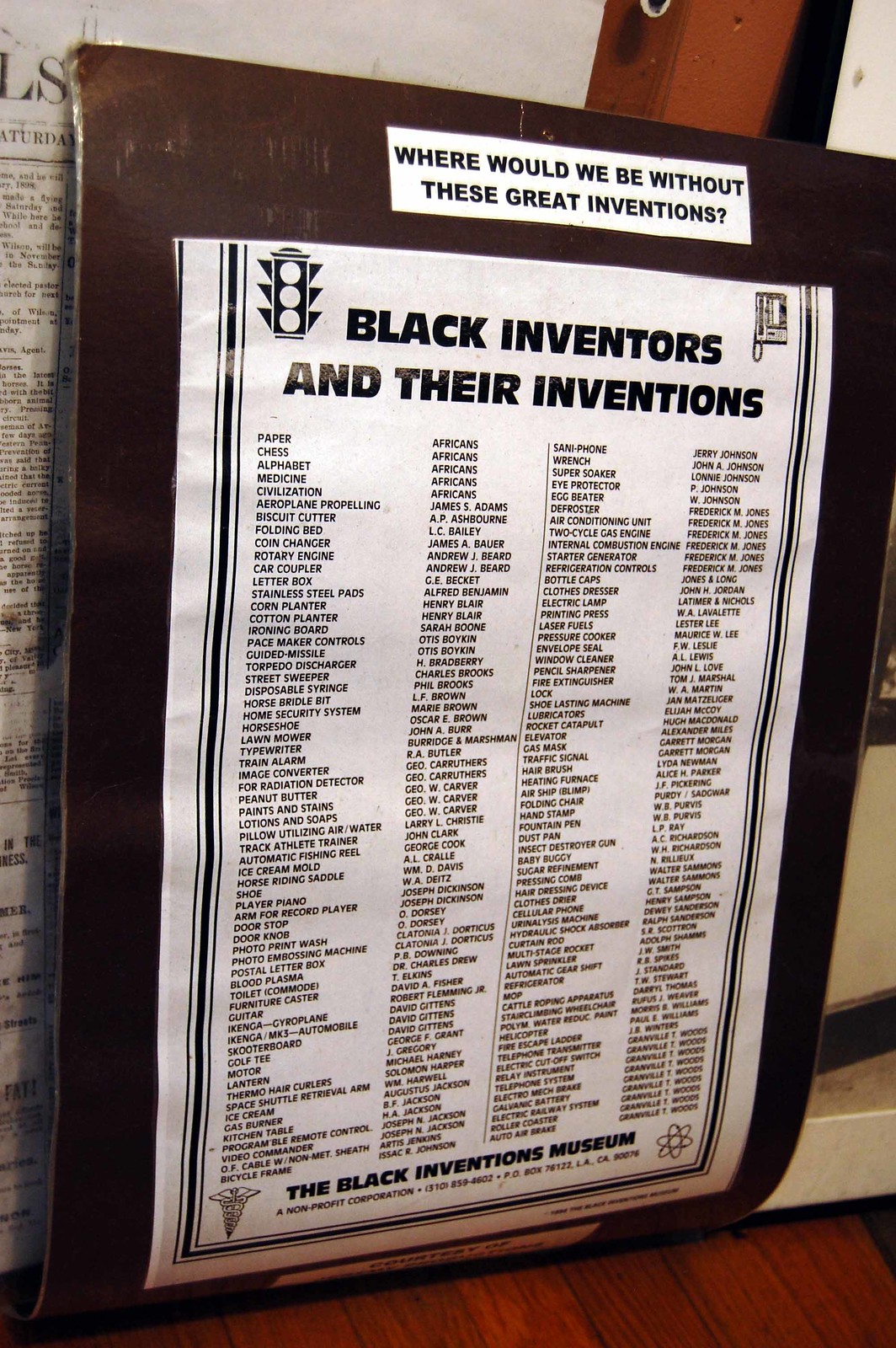The image displays a weathered, laminated brown sign, possibly glued onto a curved wooden or leather board, promoting the Black Inventors Museum in Los Angeles. At the top, encased in a white rectangle, bold black text reads, "Where would we be without these great inventors?" Directly below, another header states, "Black inventors and their inventions." Featured prominently are images of a traffic light and a phone in the upper corners. The middle of the sign is divided into four columns listing various inventions and their creators. The leftmost column details contributions credited to Africans, including paper, chess, alphabet, medicine, and civilization. Subsequent columns list specific inventions like the airplane propeller by James Adams, Sanifone, wrench, and Super Soaker, alongside names like Jerry Johnson, John A. Johnson, P. Johnson, W. Johnson, and Frederick M. Jones. The bottom of the sign advertises the Black Inventors Museum, providing contact information: a phone number (310-859-4602), and an address, P.O. Box 76122, Los Angeles, California, 90076.